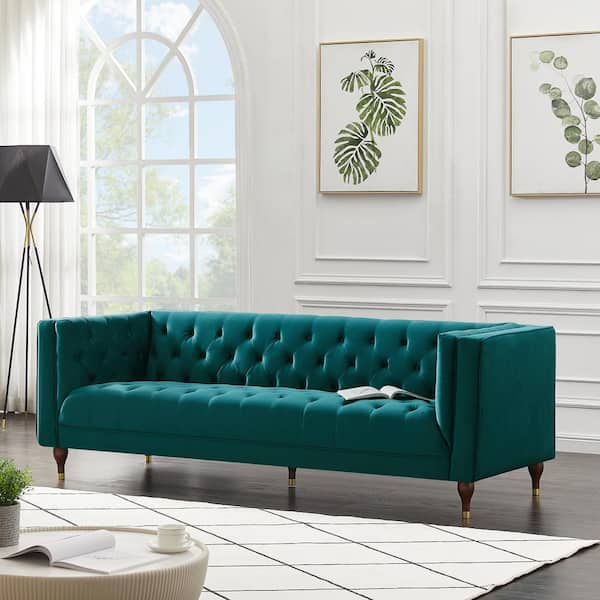The image showcases a luxurious living room with a hardwood floor. At the center of the room is a wide, teal-colored sofa with brown wooden legs, designed with visible indents. A publication, either a book or magazine, rests atop the couch. The wall behind the sofa is adorned with framed artwork featuring green leaves, including palm fronds and other leafy plants, set in gold frames with white inserts. To the left side of the image, there is a white coffee table that holds an open book, a coffee cup, and a potted plant. A white rug with black lines adds texture to the wooden floor. The living room also features white walls with classy square or rectangular molding, a black lamp next to the couch, and a large window with a white frame.